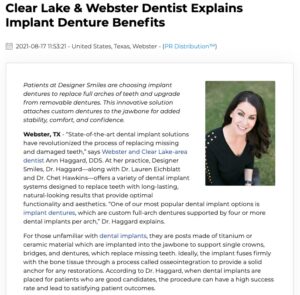This image appears to be a screenshot from a website featuring an article or advertisement about the benefits of implant dentures. The top of the image has a bold black heading that reads "Clear Lake and Webster Dentist Explains Implant Denture Benefits." Directly underneath, in gray text, is the date "2021/06/17" accompanied by a time stamp. Below that, the article is titled "United States, Texas Webinar" with some blue text beside it. The main body of the article consists of three paragraphs explaining the implant denture benefits. To the upper right of these paragraphs is a color photograph of a Caucasian woman with dark brown hair, dressed in a black blouse. The backdrop of the photo is green. The article appears to be a detailed write-up from a professional source, likely a magazine, book, or online publication.